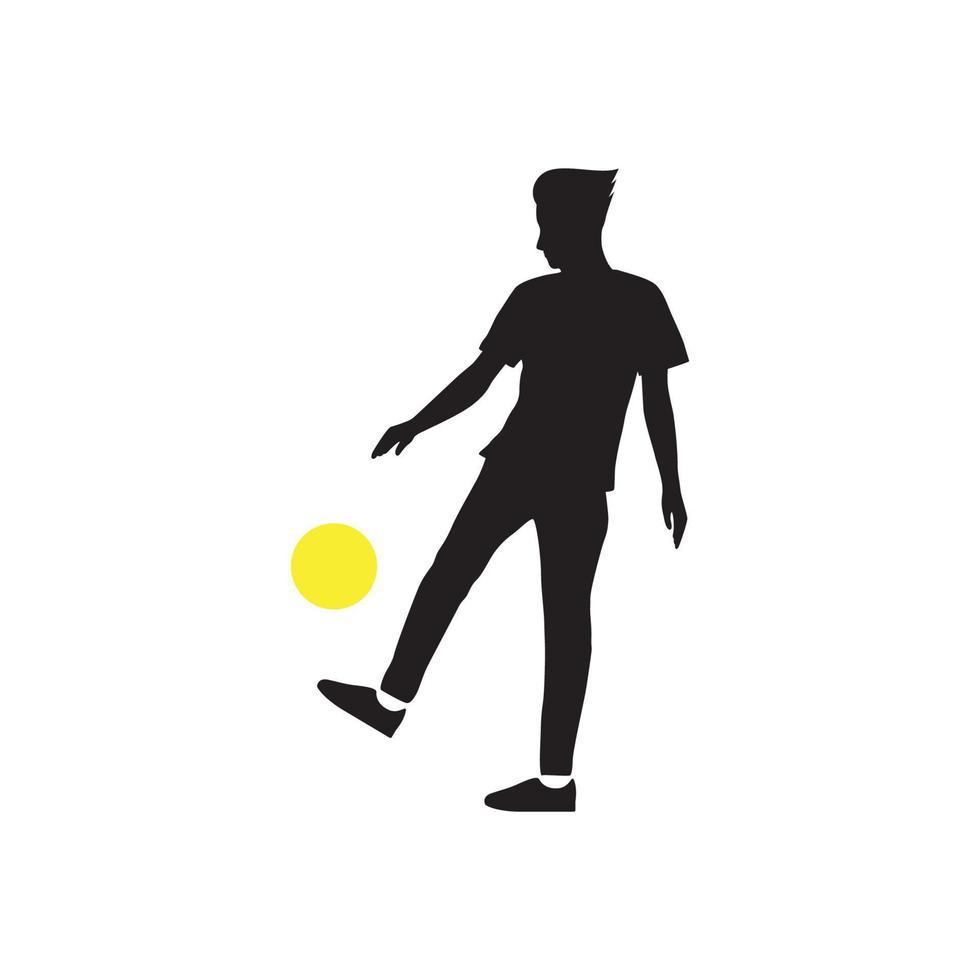The image showcases a silhouette of an adult male, depicted entirely in solid black, except for the area between his pant cuffs and black shoes, which is white. The background is white, providing a stark contrast that makes the silhouette stand out clearly. The man, dressed in a short-sleeve t-shirt and pants, is oriented with his body facing left while his head turns to the left, revealing hair that is swooped up and outward towards the right. His right leg is raised, as he is in the process of kicking a bright yellow circle, which represents a soccer ball. His arms hang naturally beside him, slightly away from his waist. The image is devoid of other colors, words, or numbers, and appears to be well-lit and clear, emphasizing the shadow-like depiction of the man.